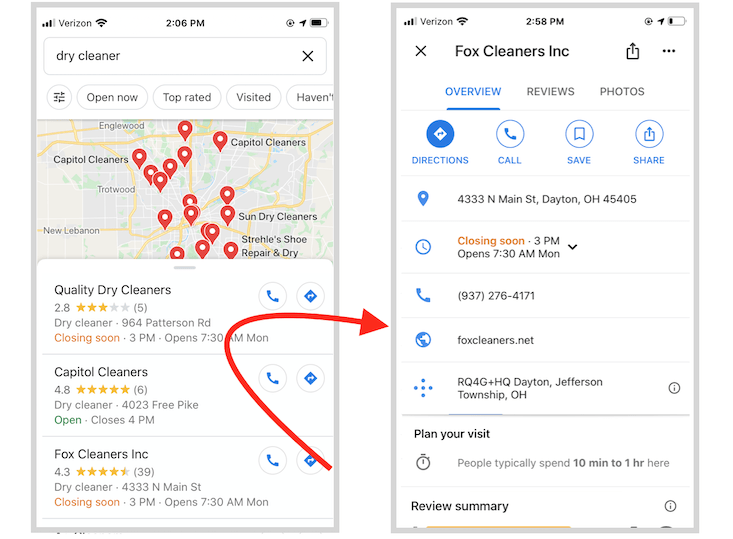Sure, here's a detailed and cleaned-up caption for the dual image:

---

**Dual Phone Screen Screenshot Comparison:**

*First Screenshot (Top Image):*

The screenshot captures the display of a smartphone, with the status bar indicating Verizon as the network provider. The signal strength shows three out of four bars, and the Wi-Fi icon appears to be fully connected. Displayed in the center is the time reading 2:06 PM. On the right side of the status bar, the battery icon is approximately three-quarters full. Adjacent to the battery icon on the left is an arrow, and a somewhat indistinct circular icon.

Below the status bar, the main content of the screen is visible, consisting of a highlighted search result for "dry cleaner" within a long rectangular field ending with an 'X' for clearing the search. Following this are several interactive buttons labeled "Open now," "Top rated," "Visited," and "Haven't." 

A map section is shown next, marked with several red location pins indicating various points of interest. Underneath the map, three sections list different dry cleaners: 
1. Quality Dry Cleaners (Rating: 2.8)
2. Capital Cleaners (Rating: 4.8)
3. Fox Cleaners (Rating: 4.3)

An arrow directs attention to the second screenshot pertaining to Fox Cleaners.

*Second Screenshot (Bottom Image):*

Mirroring the layout of the first screenshot at the top, this one shows the time as 2:58 PM. The featured highlighted search result is now specifically for "Fox Cleaners."

This screen details the profile of Fox Cleaners, segmenting the content into tabs: Overview, Reviews, and Photos. An address and phone number are provided, accompanied by relevant icons for easy navigation. Towards the bottom, there are options to "Plan your visit," followed by additional information and a "Review summary" section.

---

This revised caption provides a clear, thorough description of the dual-image screenshot, detailing each aspect for better visual comprehension.